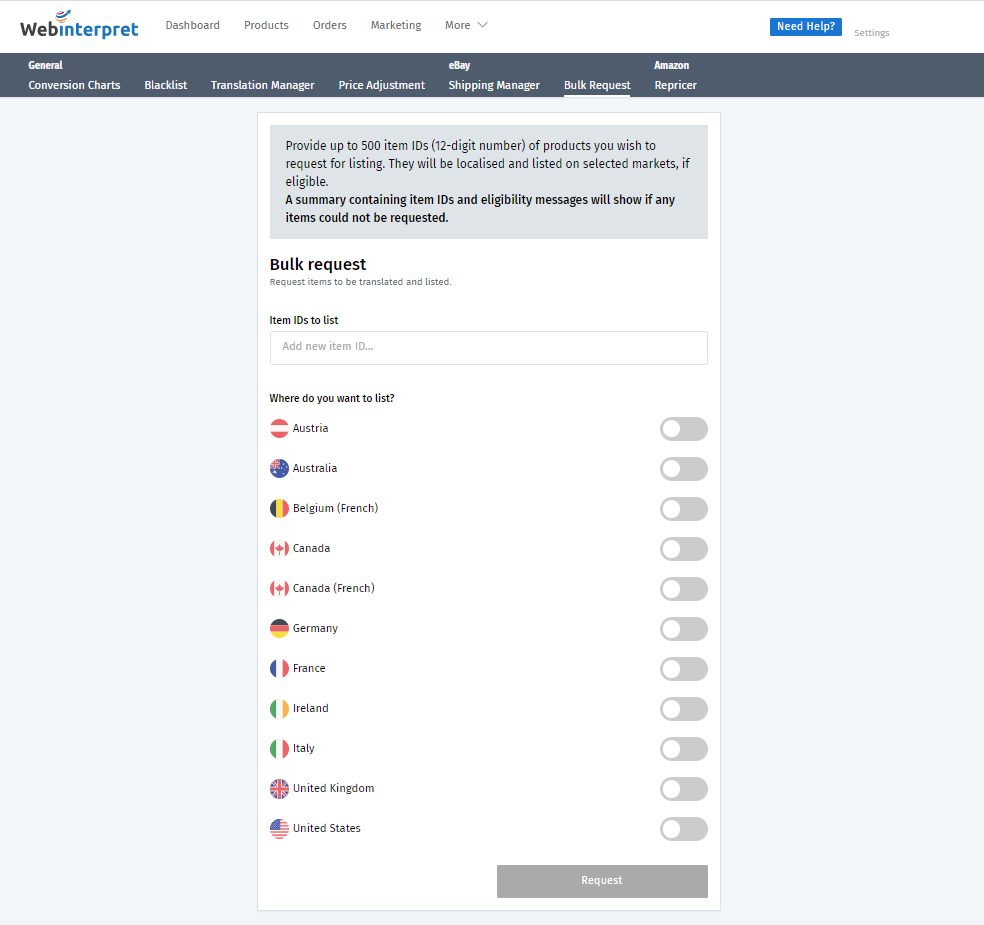This screenshot from the Web Interpret company dashboard displays a comprehensive interface for managing e-commerce tasks. At the top, it features navigation tabs including "Dashboard," "Products," "Orders," "Marketing," and more. Additionally, there are buttons for accessing help resources and settings. Below these, specific sections labeled "General," which include options like "Conversation Charts," "Blacklist," "Translation Manager," "Price Adjustments," and "Shipping Manager," can be seen.

Directly above these sections, the interface allows users to toggle between eBay and Amazon-specific settings, with options for "Bulk Request" and "Repricing." The main part of the screenshot centers on a user action area designed for listing products. Here, users can select their desired markets from countries including Austria, Australia, Canada, Germany, Ireland, Italy, and the United States, by using toggle buttons next to each country’s name.

In the main action section, users are prompted with the question, "Where do you want to list?" indicating the feature is tailored for sellers who wish to list items across different countries. Users are instructed to provide up to 500 item IDs, represented as 12-digit numbers, for the products they wish to list. These products will then be localized and listed on the selected markets. This detailed setup enables sellers to manage their product listings efficiently across different international e-commerce platforms.